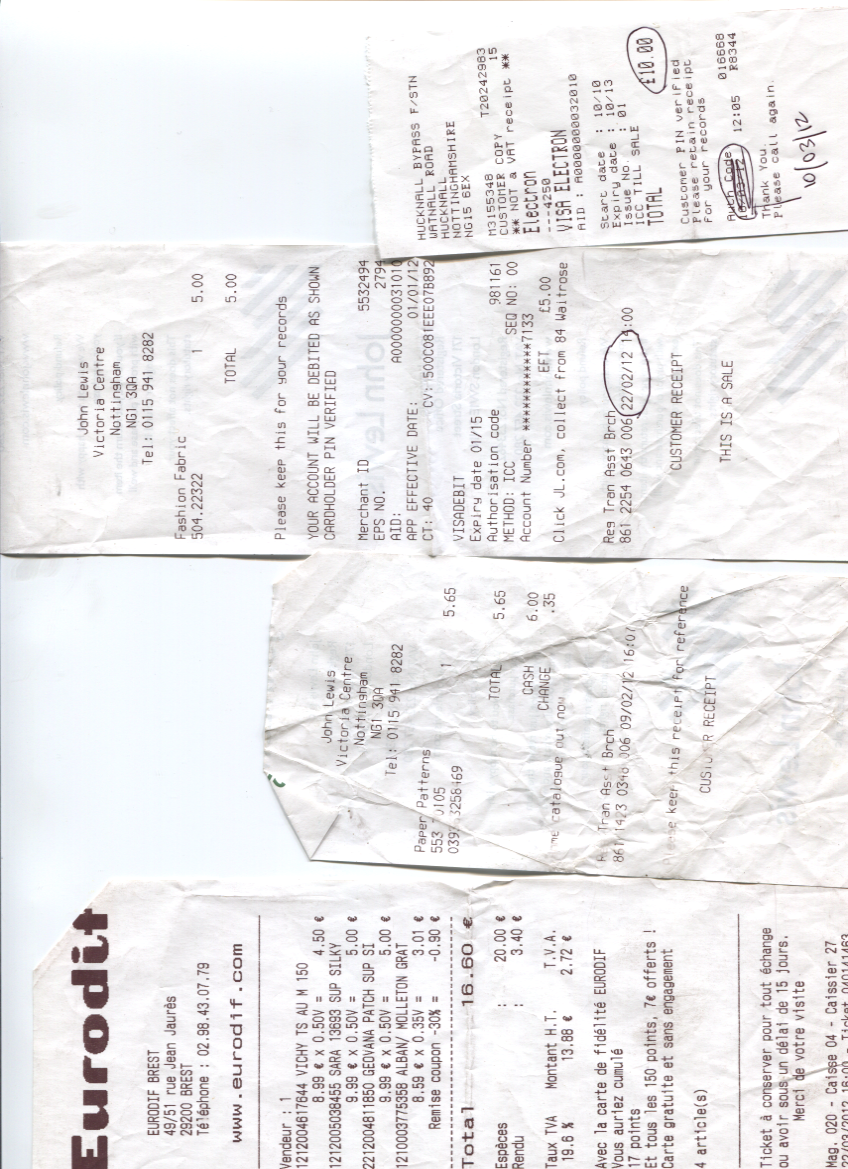The image depicts a photograph of four retail receipts placed against a white background, likely taken with a cell phone. Each receipt displays detailed transactions, complete with item lists, total costs, and the retailer's name at the top. One receipt features a circled amount of £10, while another highlights a date circled '2022-02-12'.